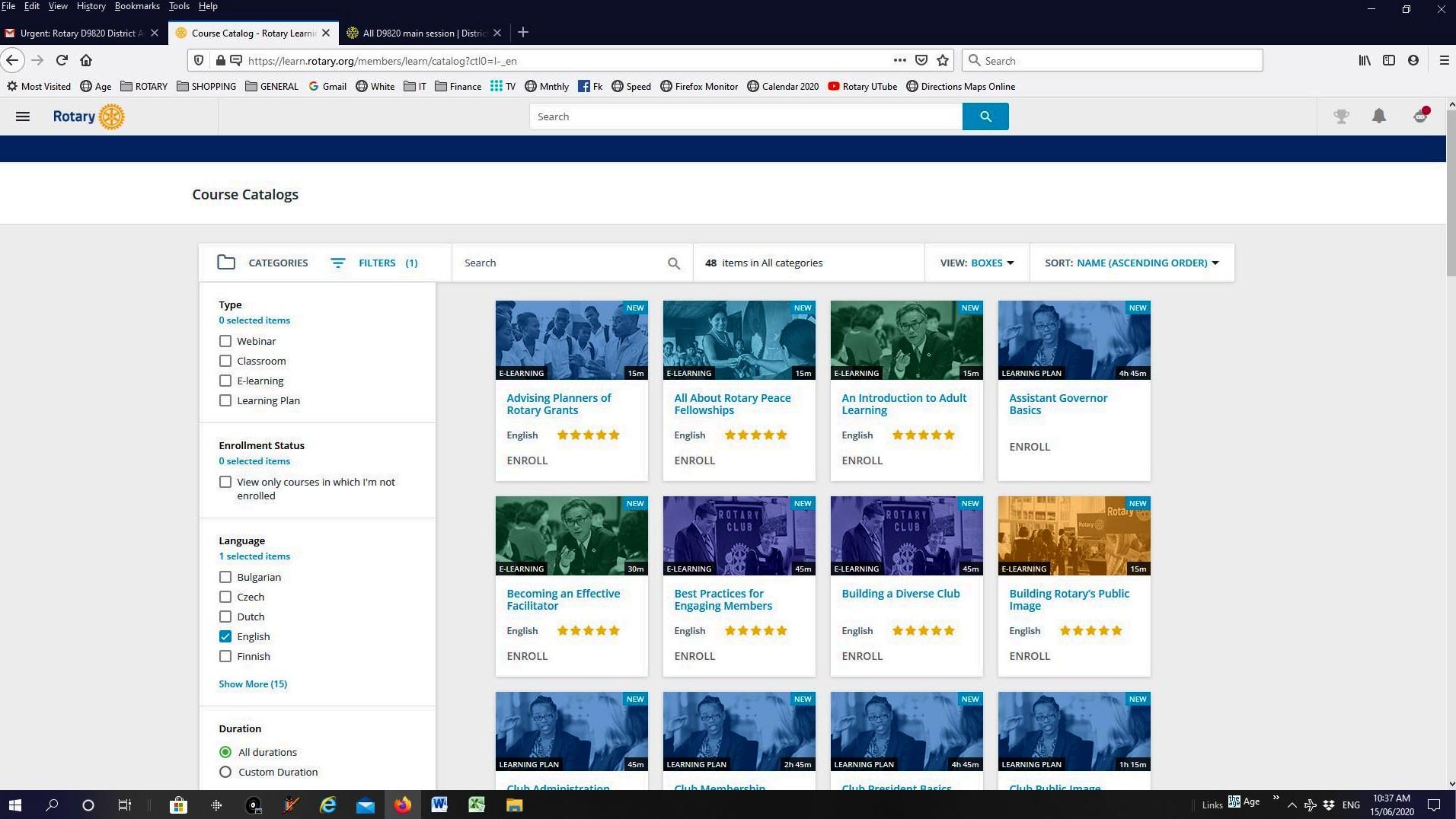### Screenshot of Rotary Learning Website

This screenshot captures the interface of a web browser window displaying the Rotary Learning website. 

**Top Bar:**
- In the upper left corner, standard menu options are visible: "File," "Edit," "View," "History," "Bookmarks," "Tools," and "Help."

**Tabs Bar:**
- Below the main menu, the tabs bar features three tabs:
  1. "Urgent Rotary D 9820 District" (partially visible),
  2. The highlighted tab titled "Course Catalog - Rotary Learning,"
  3. "All D 9820 Main Session."

**Address Bar:**
- The URL in the address bar is: "http://learning.rotary.org/member/learn/catalog."

**Menu Bar:**
- Directly underneath the address bar, a toolbar with assorted icons and labels extends from left to right:
  1. A sprocket icon labeled "Most Visited,"
  2. A world icon labeled "Age,"
  3. A folder icon labeled "Rotary,"
  4. A photo icon labeled "Shopping,"
  5. A folder icon labeled "General,"
  6. A Gmail button,
  7. Another world icon labeled "White,"
  8. A folder icon labeled "IT,"
  9. A folder icon labeled "Finance,"
  10. A TV button,
  11. A "Monthly" button,
  12. A Facebook button,
  13. A "Speed" button,
  14. A Firefox monitor button,
  15. A "Calendar 2020" button,
  16. A "Rotary YouTube" button,
  17. A "Directions Map Online" button.

This detailed description encapsulates the key visual elements of the screenshot, highlighting the structure and contents of the Rotary Learning website interface as displayed within a web browser.